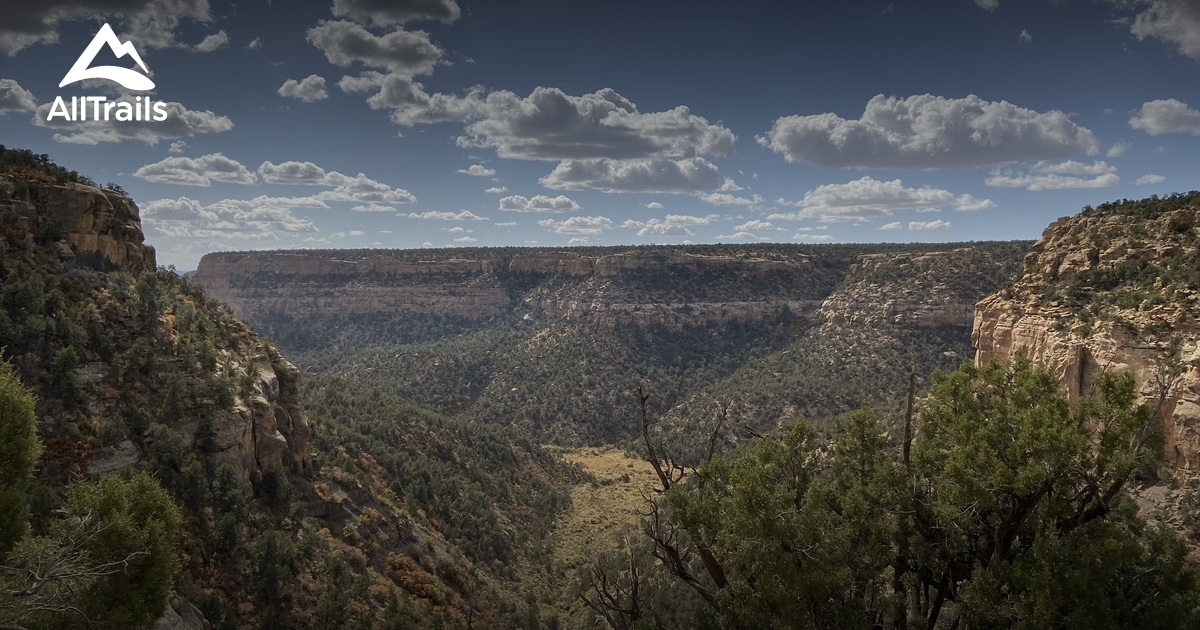The image depicts a rugged canyon landscape, likely reminiscent of the Grand Canyon, showcasing dramatic cliffs and a descending canyon floor. The foreground features a tree with pine needles and some dead branches, situated in the bottom right corner. The center of the image reveals the canyon's floor, leading up to hillsides and imposing rock bluffs that culminate in flat-topped cliffs. On the right side, behind the mentioned tree, another cliff adds to the layered depth of the scene. The bottom left corner shows more cliffs adorned with trees and bushes. The sky above is a hazy blue, filled with fluffy white clouds, suggesting a sunny day. In the top left corner, a white logo of a mountain symbol accompanies the text "All Trails," indicating the image is part of an advertisement, likely for the All Trails app, designed for hiking enthusiasts. The colors in the image range from blue and white in the sky to the tans, browns, and greens of the canyon and its sparse vegetation, which consists mainly of evergreen trees, shorter shrubs, and scattered bushes.